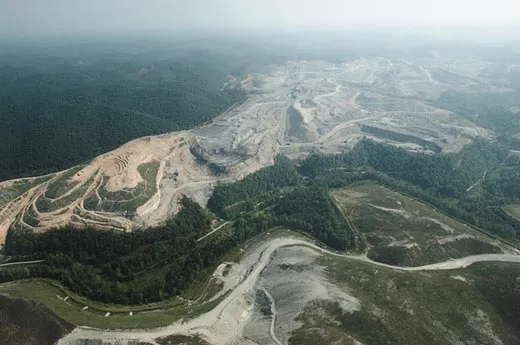An aerial photograph captures a mountainous landscape enveloped in fog and an overcast sky, creating a mysterious and somewhat hazy atmosphere. The photograph, likely taken at around 1,000 feet, showcases a mountain range with varying terrain. At the left side of the image, there's a quarry and a dense forest that extends across the upper left and down to the bottom of the mountains. The middle section of the photo features a series of winding trails that crisscross up and around the mountains. The mountain itself appears flat-topped and could be either snow-capped or covered in white sand-like material.

The scene includes both forested and non-forested areas, with the latter covered in grass. There is a notable bright light source, but due to the foggy lens, the finer details are obscured. In the background, additional mountainous formations are faintly visible.

In the foreground, scattered man-made structures and a winding road can be seen, blending into the natural landscape. The right side of the image tends towards a gray-brown hue, possibly indicating sandy or barren land, which contrasts with the clearer, more detailed forested region to the left. The coastline-like edge towards the far right is indistinct, adding to the overall enigmatic quality of the photograph.